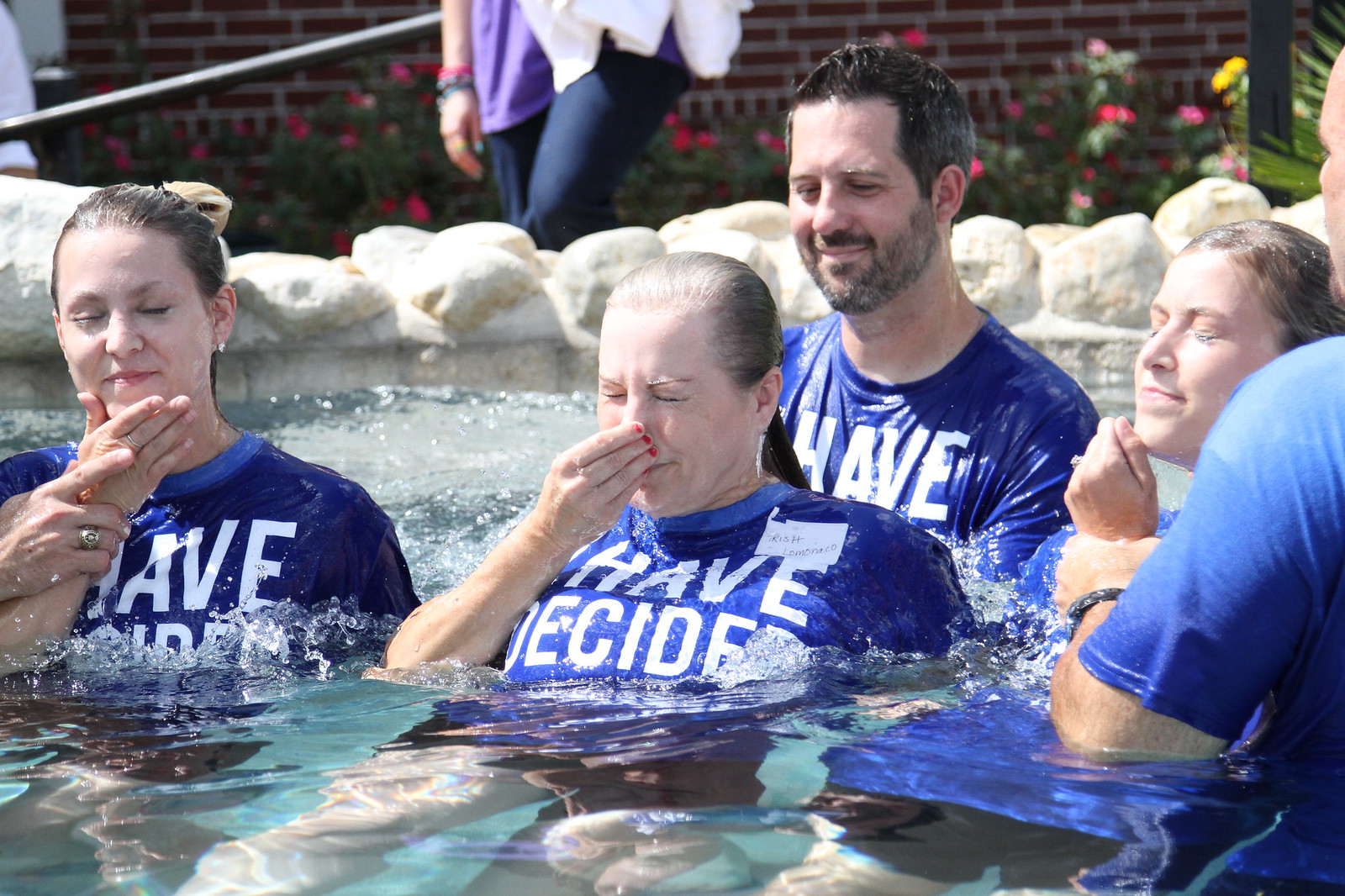In this image, a group of five people—a man and four women—are gathered in a small, clear pool surrounded by a rocky border. All five individuals are wearing blue shirts emblazoned with the phrase "I have decided," suggesting a religious theme, likely a baptism. The man stands behind the women, gently supporting the woman in the middle, who has her nose pinched, indicating she might be submerging or surfacing from the water. The other women are either holding their noses or chins, and all appear to be smiling and content. Behind the pool, a brick wall adorned with bushes and flowers creates a pleasant backdrop. A woman can be seen walking along this wall, reinforcing the serene, communal atmosphere of the scene.